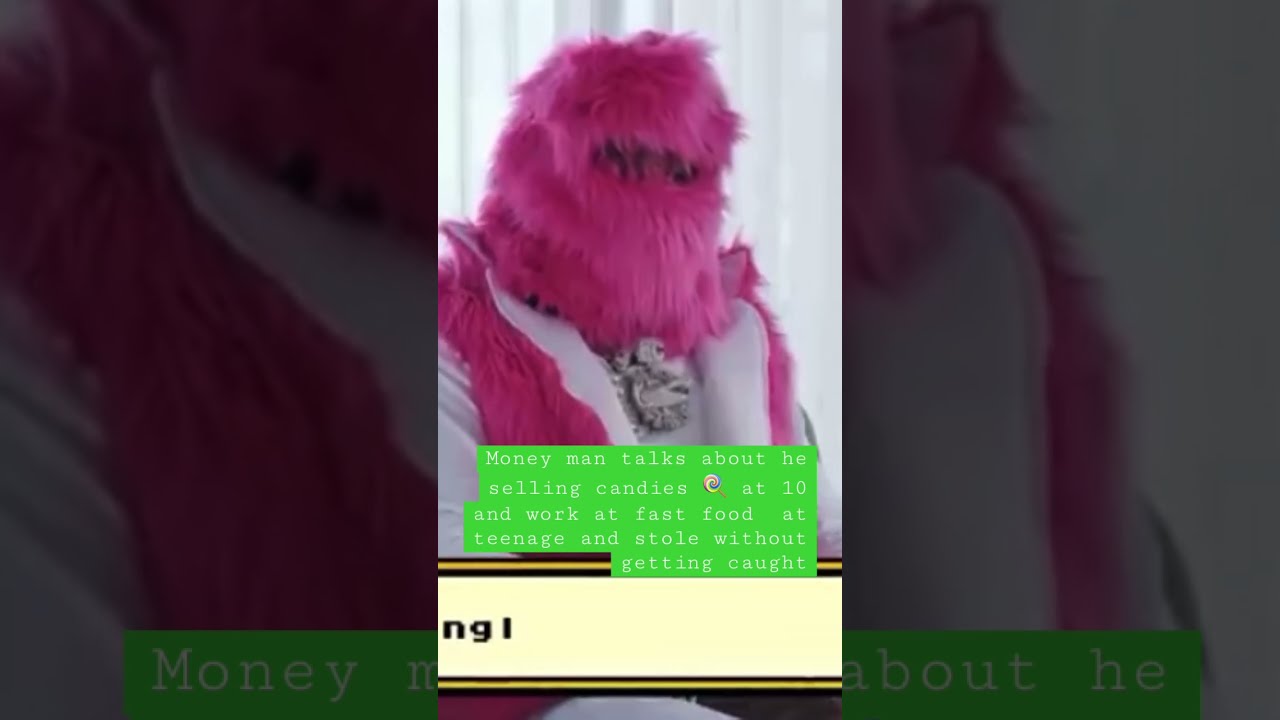The image is divided into three vertical sections, with the first and third sections containing darkened, close-up versions of the central image. The central section features a person in a costume, consisting of a fluffy, pink, and furry headpiece and torso piece, set against a white background. The costume covers the individual's face, leaving only black eyes visible. They appear to be wearing a white shirt and a large, obscure necklace.

The background of the central image is a faded, larger version of itself. Below the central figure, there is a green rectangle with white text. The text reads: "Money Man talks about selling candies at 10, working at fast food as a teenager, and stealing without getting caught." The overall appearance suggests an advertisement or promotional material.